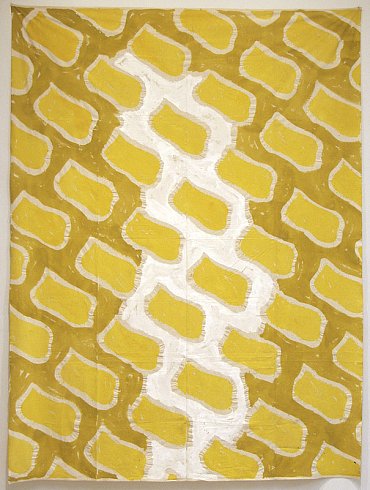The image depicts a rectangular piece of art with a thin gray border that extends all around the frame. The main background is a dark yellow color, featuring rows of lighter yellow brick-like shapes outlined in gray. These bricks are arranged diagonally, slanting upwards across the entire canvas. Centrally, there is a prominent vertical column of white, extending approximately 90% of the way up from the bottom. The white section brings to mind abstract imagery, possibly resembling an upright figure. This composition, somewhat reminiscent of a fabric pinned to a wall by its top corners, also includes an overall tone where the background outside the main dark yellow area is an off-white color.